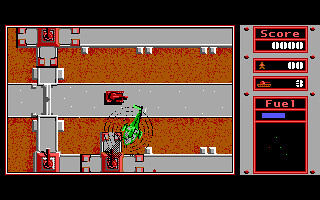The image is a small, rectangular, color display from a retro video game, framed by black borders at the top and bottom. The game's background is pixelated, featuring an old-style digital display dominated by orange and red colors, simulating a surface speckled with red and brown. In the game's center left, there are horizontal gray and orange walkways resembling roads with white speckles. Toward the bottom left, two characters stand: one in gray and another in green. Scattered across the walkways are red vehicles, including a red tank on the middle road with its cannon pointed right, and two other red tanks moving vertically up the screen. A green helicopter with black circles around it, representing moving blades, is also present. 

Toward the left side, a gray robot-shaped figure is visible. To the right side of the screen, a panel displays game information with black rectangles outlined in red. The scoreboard reads "Score 0000" in red and white letters, with additional stats below it: a person's score marked as "00," three tanks indicated, and a fuel gauge with a nearly full blue bar. The panel ends with an empty black box underneath.